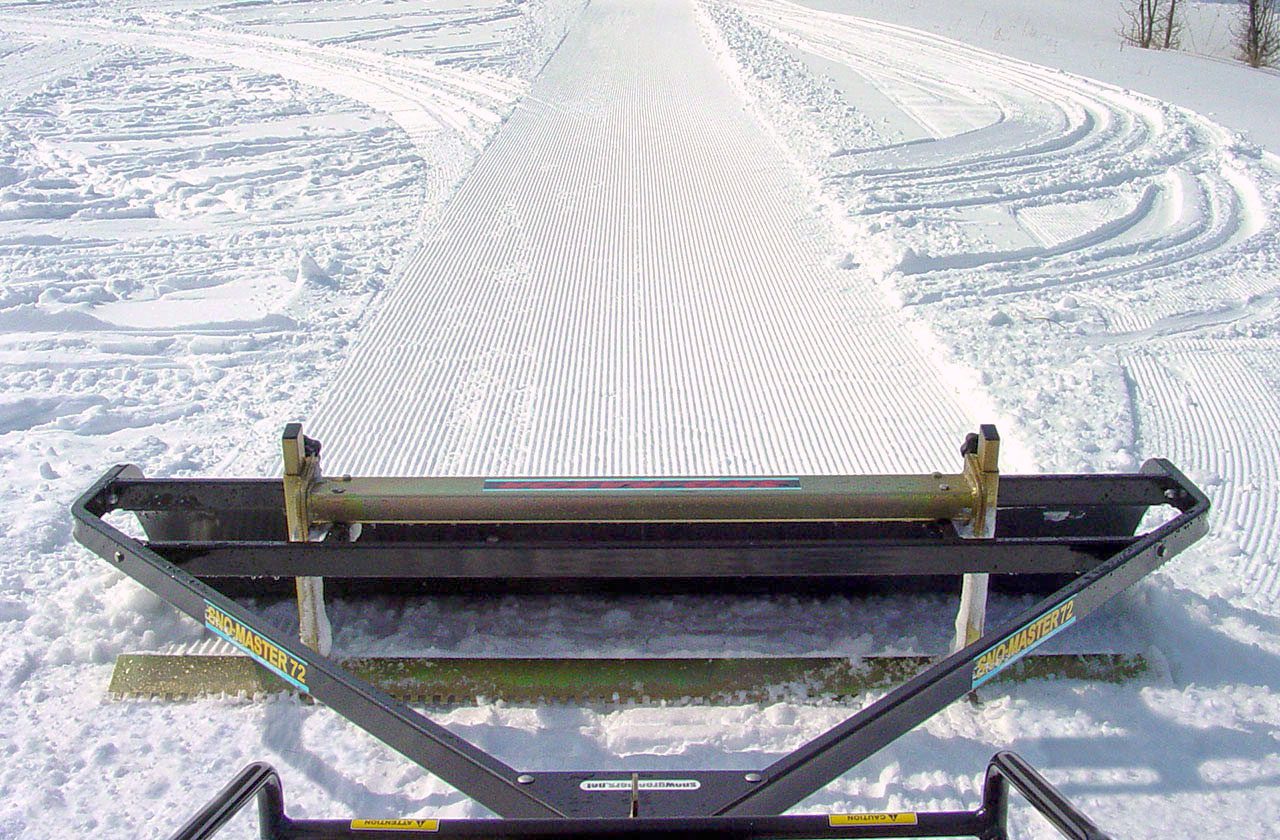This photograph captures a winter scene featuring a large, snow-covered field with numerous circular tire tracks around its edges. The main focus of the image is a silver, metal-colored snow plow situated at the bottom, with tracks indicating its path through the center of the snow field. The snow plow is smoothing out the snow, leaving behind intricate grooves and a flattened, even surface, as it is dragged along possibly by another vehicle. The background includes two trees, hinting at an outdoor setting, potentially someone's backyard, a park, or a ski slope being prepared for use. The vivid white snow contrasts with the dark, metallic hue of the snow plow, and the scene is likely captured in a real-life photo taken with a smartphone.